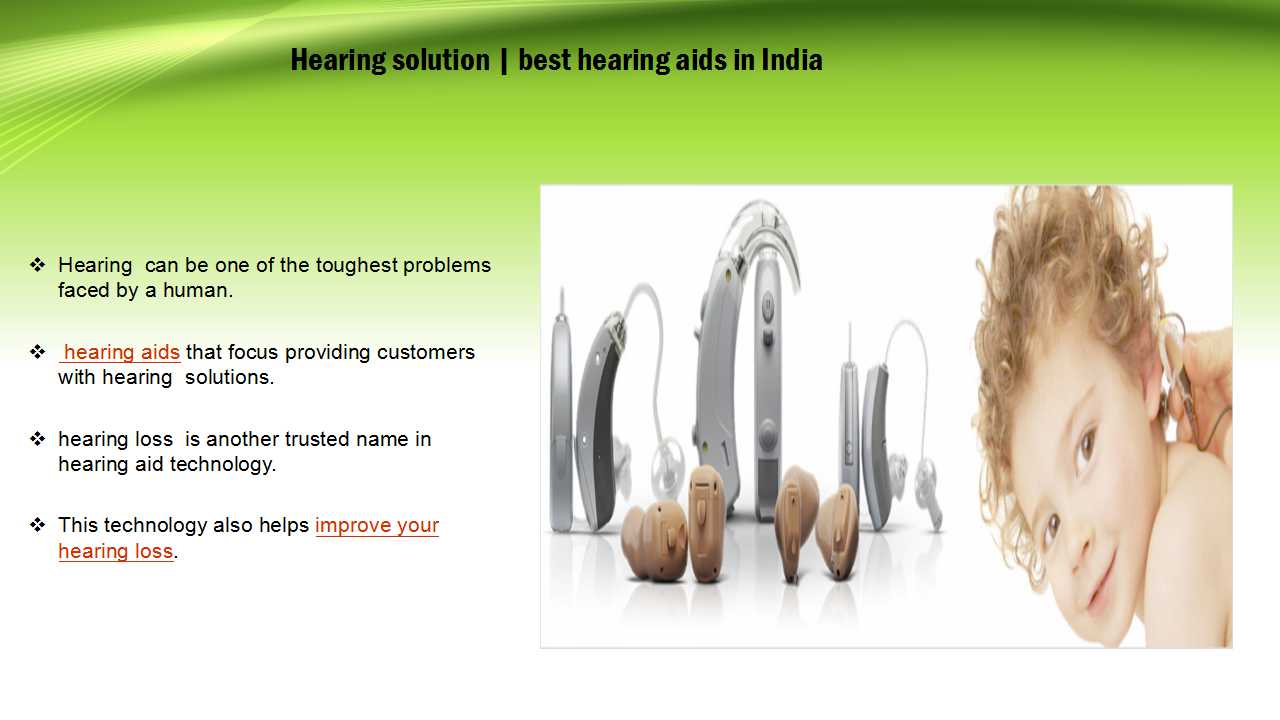This informative advertisement for hearing aids, particularly targeting children in India, features a mix of images and text. At the top of the ad, a lime green banner displays in black lettering: "Hearing Solutions / Best Hearing Aids in India." Below this, there are four bullet points conveying key messages: 
1. "Hearing can be one of the toughest problems faced by a human."
2. "Hearing aids that focus on providing customers with hearing solutions."
3. "Hearing loss is another trusted name in hearing aid technology."
4. "This technology also helps improve your hearing loss" (with "hearing aids" and "improve your hearing loss" highlighted in red and underlined). 

To the right, set against a white background, are images of various hearing aid models. In the foreground is a young child, possibly three or four years old, with light, dirty brown curly hair. The child is looking down with a slight smile as a doctor touches his ear, showcasing the hearing aid.